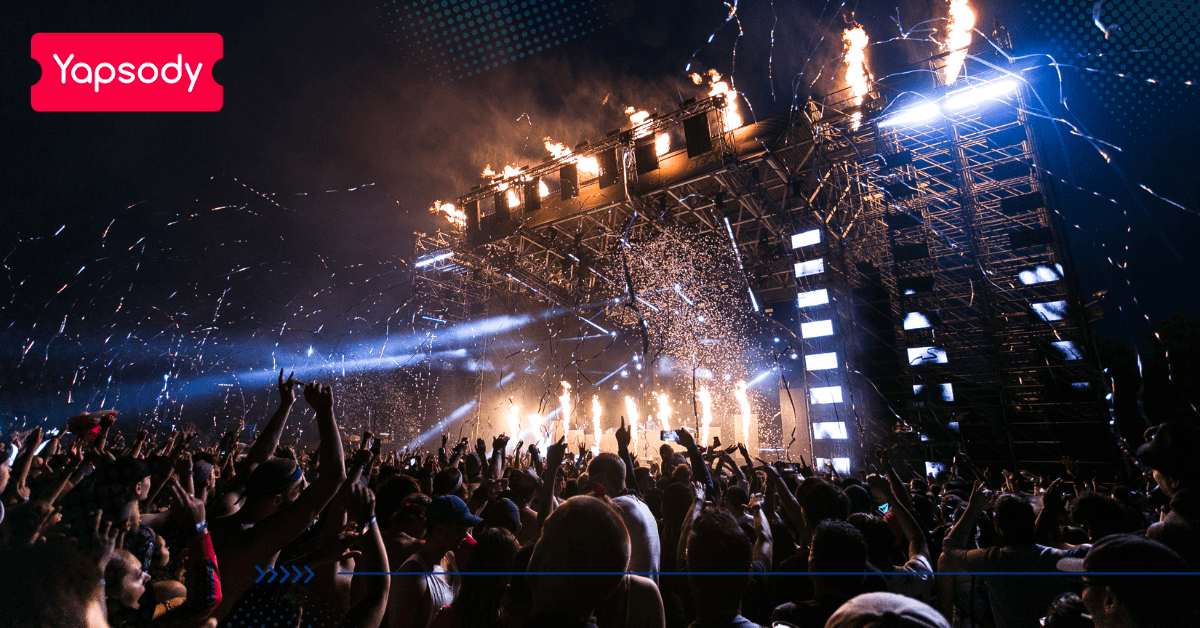The image captures an electrifying night-time rock concert with an expansive, metal-structured stage as its centerpiece. Brilliant pyrotechnics light up the scene, with flames shooting both on and above the stage, creating a dramatic effect. The atmosphere is further energized by blue strobe lights that cut through the darkness, illuminating the sea of excited fans. Hands are raised high in the air, with many attendees snapping photos or gesturing enthusiastically. The crowd mostly wears dark clothing, blending into the night backdrop. In the upper left corner, a red ticket stub-shaped icon prominently displays the text "YAPSODY" in white letters, indicating this might be a promotional image for the event.